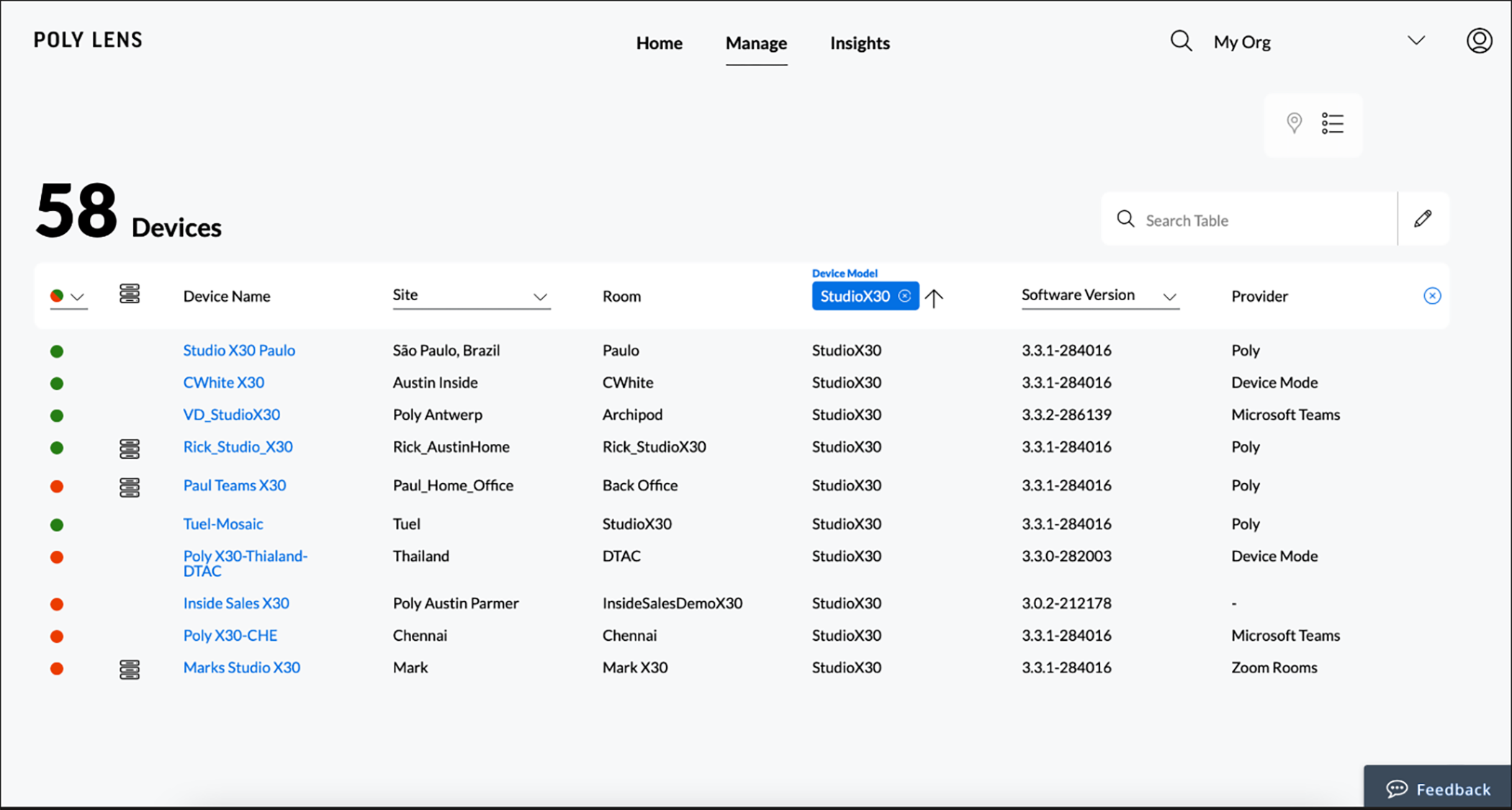This screenshot captures the detailed layout and interface of a management page from the Poly Lens platform. The background is a light gray shade, creating a soft and professional backdrop.

In the upper left-hand corner, the text "Poly Lens" is prominently displayed. Centered at the top are three navigational categories: Home, Manage, and Insights, with the "Manage" category underlined to indicate the current page view. Towards the upper right-hand corner are a search icon, the label "My Org," and a drop-down menu.

Directly beneath this top row is a filter button. Below that, aligned to the left, is a large, bold number "58" followed by the label "Devices." On the same row to the right, there is a search bar labeled "Search Table" and an Edit button.

The table below features a white header. The columns in this header include several distinctive attributes:
- The first column contains a status indicator (either a green or red circle) coupled with a drop-down menu.
- An icon resembling three stacked rectangles with rounded tops.
- "Device Name" labeled with an underline and a drop-down menu.
- "Site," also with an underlined label and a drop-down menu.
- "Room."
- The next column starts with a blue button labeled "Studio X 30," indicating the device model with an up arrow.
- "Software Version," underlined with a drop-down menu signaled by a down arrow.
- "Provider," which includes an 'X' button that is blue, allowing users to clear this column content.

This comprehensive interface showcases the meticulous structure and user-friendly design intended for managing devices within the Poly Lens platform.